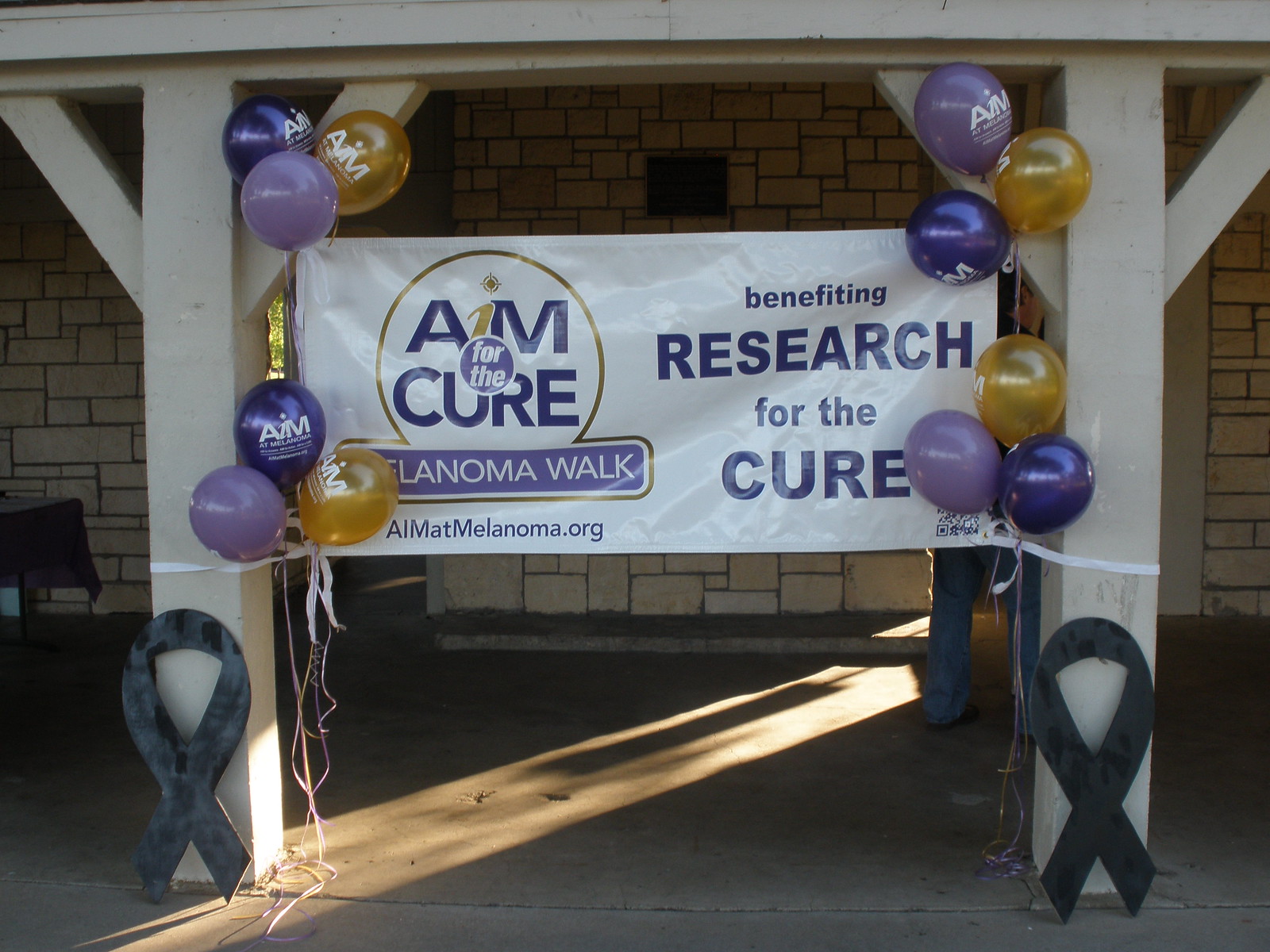In this image, we see a well-organized outdoor setting for a melanoma charity walk, highlighted by a prominently displayed banner with the message, "Aim for the Cure, Melanoma Walk" and the URL "aimatmelanoma.org," promoting research for a cure. The banner has a white background adorned with text in shades of blue, purple, and gold, specifically noting that the letter "I" in "aim" is golden. 

The banner is creatively suspended at the center of the image, securely tied to tan pillars on both sides. Surrounding the banner are colorful balloons in hues of dark purple, light purple, and gold, positioned at the top right, top left, bottom left, and bottom right corners. Additionally, there are black metal ribbons leaning against the base of the pillars on both sides.

The setting is defined by a tan brick wall occupying the top two-thirds of the background, juxtaposed against a gray concrete floor that constitutes the bottom third. The scene effectively captures the essence of an outdoor melanoma walk event, with the detailed and vibrant decorations adding to the sense of purpose and community spirit.